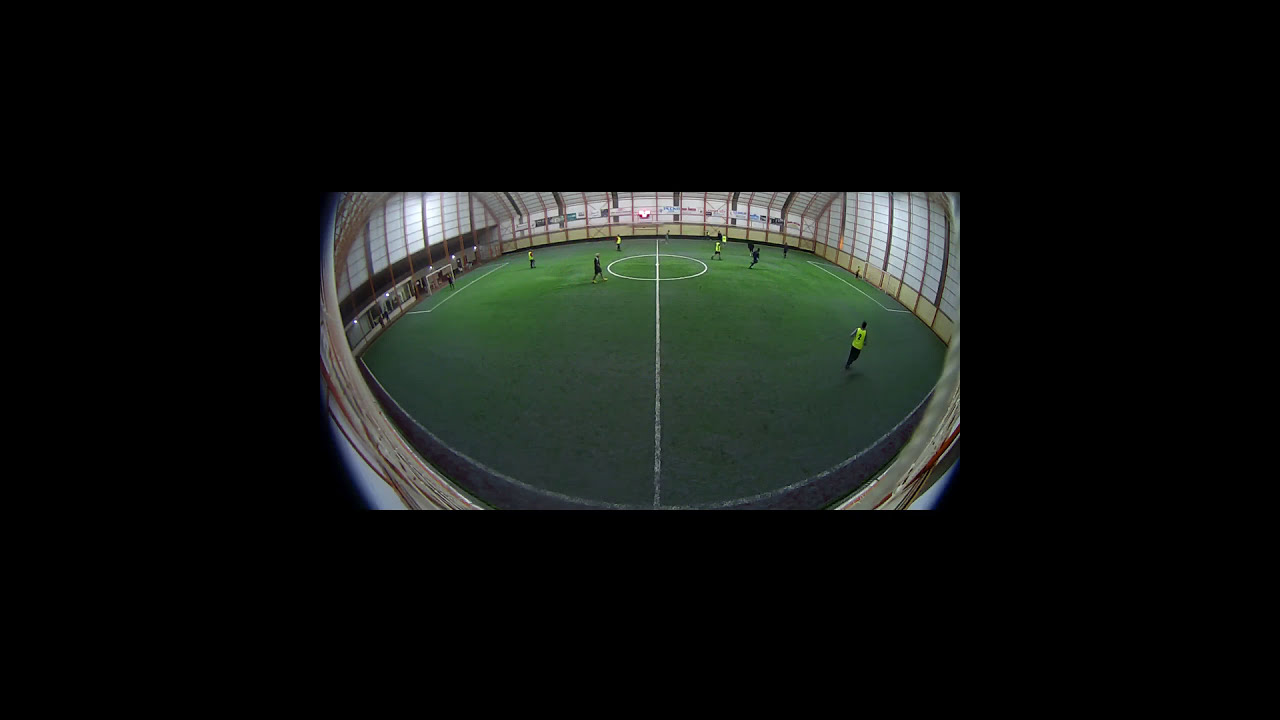The image is a horizontally aligned rectangle, dominated by a solid black background. At the center lies a smaller horizontal rectangle featuring a wide-angle, fisheye lens shot of an indoor soccer field. The green AstroTurf field is marked with typical soccer lines, including a vertical white line running through the center and a white circle at the line's midpoint. Goals are positioned at both ends of the field. The photo captures the scene from a high vantage point, likely from the top of a stadium or dome, causing the players to appear very small and the image to have a curved, distorted appearance.

In the game, a total of eight players are visible, likely in a four-on-four match. The team in bright yellow jerseys with black shorts stands out clearly, while the opposing team appears to be in dark blue uniforms, though details are indistinct due to the low resolution. Around the field are translucent panels that let light through, and sponsorship logos adorn the far wall. The high angle and low quality make it difficult to see the ball and finer details of the players.